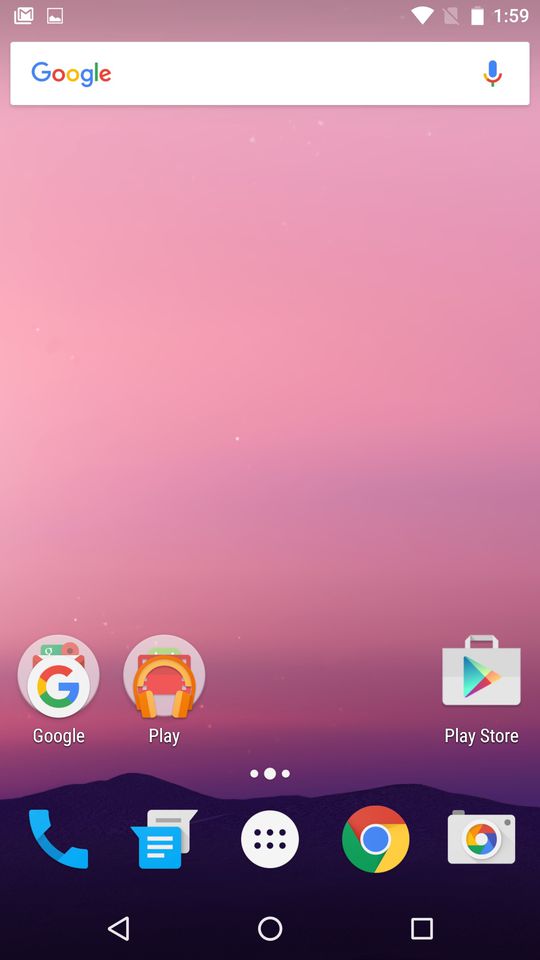This is an image of a mobile phone screen displaying the time as 1:59 PM. The device has a full battery charge and a strong network connection, both indicated at the top of the screen. At the top-center, there is a search bar with the word "Google" in its distinctive multicolored logo: a blue 'G', red 'o', yellow 'o', a lighter blue 'g', a green 'l', and a red 'e'. To the right of the Google logo, there is a small microphone icon indicating voice search functionality.

At the bottom of the screen, several app icons are displayed. The first icon, featuring a white 'G' set against a colorful background, represents the Google app. Next to it, a gray circular icon labeled "Play" is shown, with what appears to be a stylized image of orange and red earphones. Adjacent to this is the Play Store icon, depicted as a multicolored triangle within a suitcase. Also present are standard icons for phone calls (a blue phone), messaging (a blue speech bubble), and a white circle containing six black dots, typically indicating the app drawer. Finally, there are icons for Chrome, with its familiar red, green, blue, and yellow design, and Google Photos, which features a central circular motif surrounded by colored segments resembling a flower.